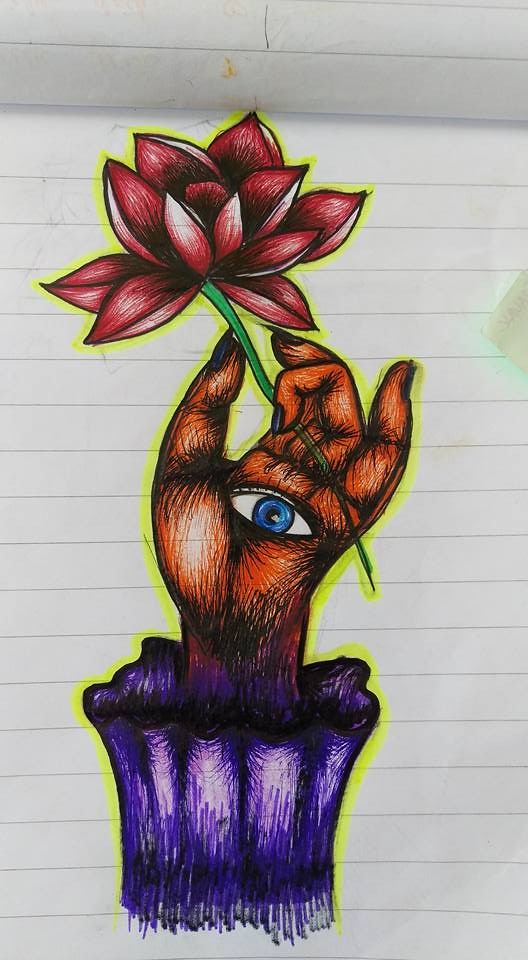The artwork, meticulously drawn on a piece of notepad paper, is primarily outlined in black ink and surrounded by a yellow highlighter border. The drawing features a dark-colored hand, likely representing a black person, adorned with blue nail polish, suggesting a feminine touch. An eye with a blue iris and black pupil, complete with eyelashes, is intricately drawn in the center of the palm. Emerging from the bottom of the image is a sleeve or jacket in shades of purple and blue. The hand, rising upwards towards the center, grasps a delicately thin green-stemmed flower with vibrant red petals. The overall image includes additional details like the cream white circle on the right side and the previous notepad page's remnant orange smudge and black line at the top, captured through the translucent paper. Horizontal black lines from the notepad paper and slight brown-black scratch details on the hand emphasize the artistic texture.